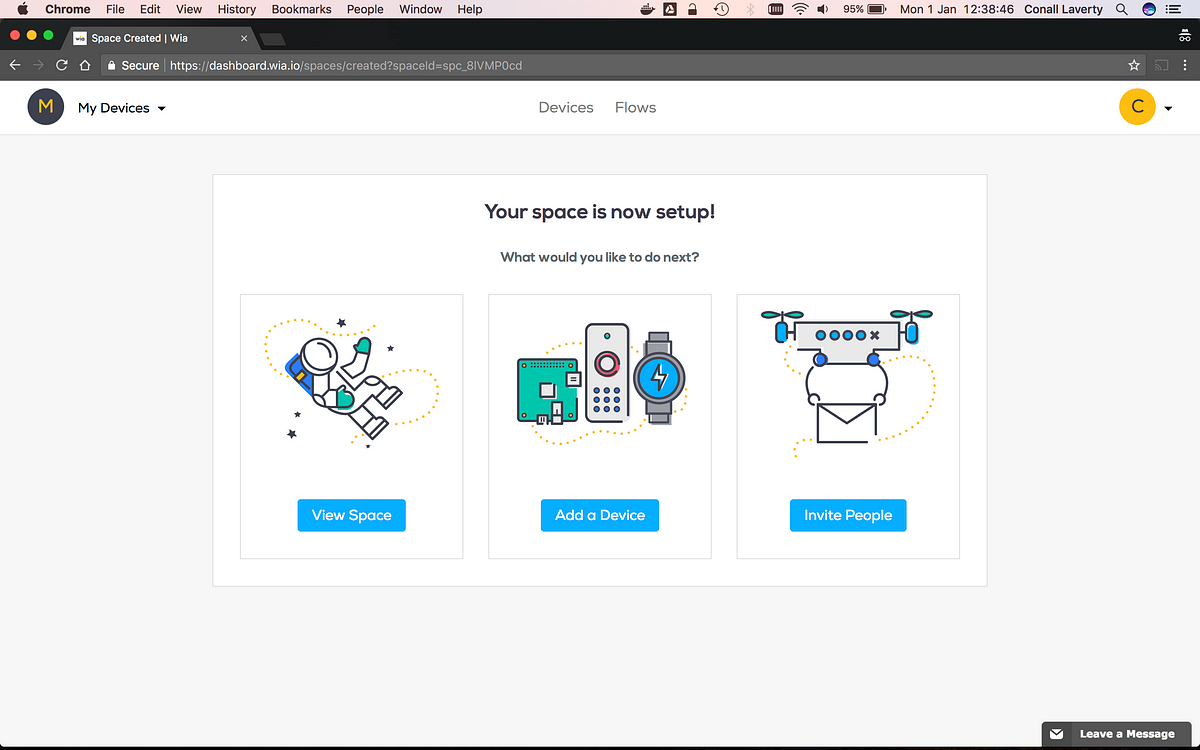This image is a detailed screenshot of a webpage, likely captured on a computer. At the very top of the screen, the Apple logo is prominently displayed in black, featuring its iconic bitten appearance. The top menu bar indicates various options such as "File," "Edit," "View," "History," "Bookmarks," "People," "Window," and "Help," alongside connectivity symbols showing online status, signal strength, and battery life, suggesting this could be a screenshot from a desktop or a laptop.

The date and time indicated are Monday, January 1st, at 12:38:48. Below this, the word "Connall Leverty" is visible alongside a diagonal magnifying glass icon for search functionality. An open browser tab, colored gray, reads "space created," followed by a vertical line and the initials "WIA."

Below this, it indicates a secure connection with the web address "dashboard.WIA.io." The background of the main content area is white. In the top left-hand corner, there's a blue circle with a yellow "M" inside it, next to the text "My Devices" in black font, accented with a downward-pointing arrow, indicating a dropdown menu.

Centered on the page, in lighter gray font, it reads "Devices," next to the word "Flows." On the right, another circular icon features a yellow background with a thin black "C," also hinting at a dropdown menu. A thin gray line separates these sections from the rest of the content.

Below this, a larger text box with a darker black font announces, "Your space is now set up!" followed by a line in smaller font asking, "What would you like to do next?"

This prompt is followed by three picture options. The first depicts a silhouette of an astronaut floating in space against a starry background. Below, a rectangular blue button with white text reads "View Space." The second image, in the middle, showcases animated objects: a computer screen on the left, a remote control in the center, and a watch on the right. Beneath these, the text reads "Add Device."

The third image, on the right, illustrates a computerized drone with two propellers, each on one side, holding an envelope. Below, it says "Invite People."

Overall, the screenshot appears to be from a user interface designed for managing devices and spaces, with interactive options for viewing, adding devices, and inviting others.